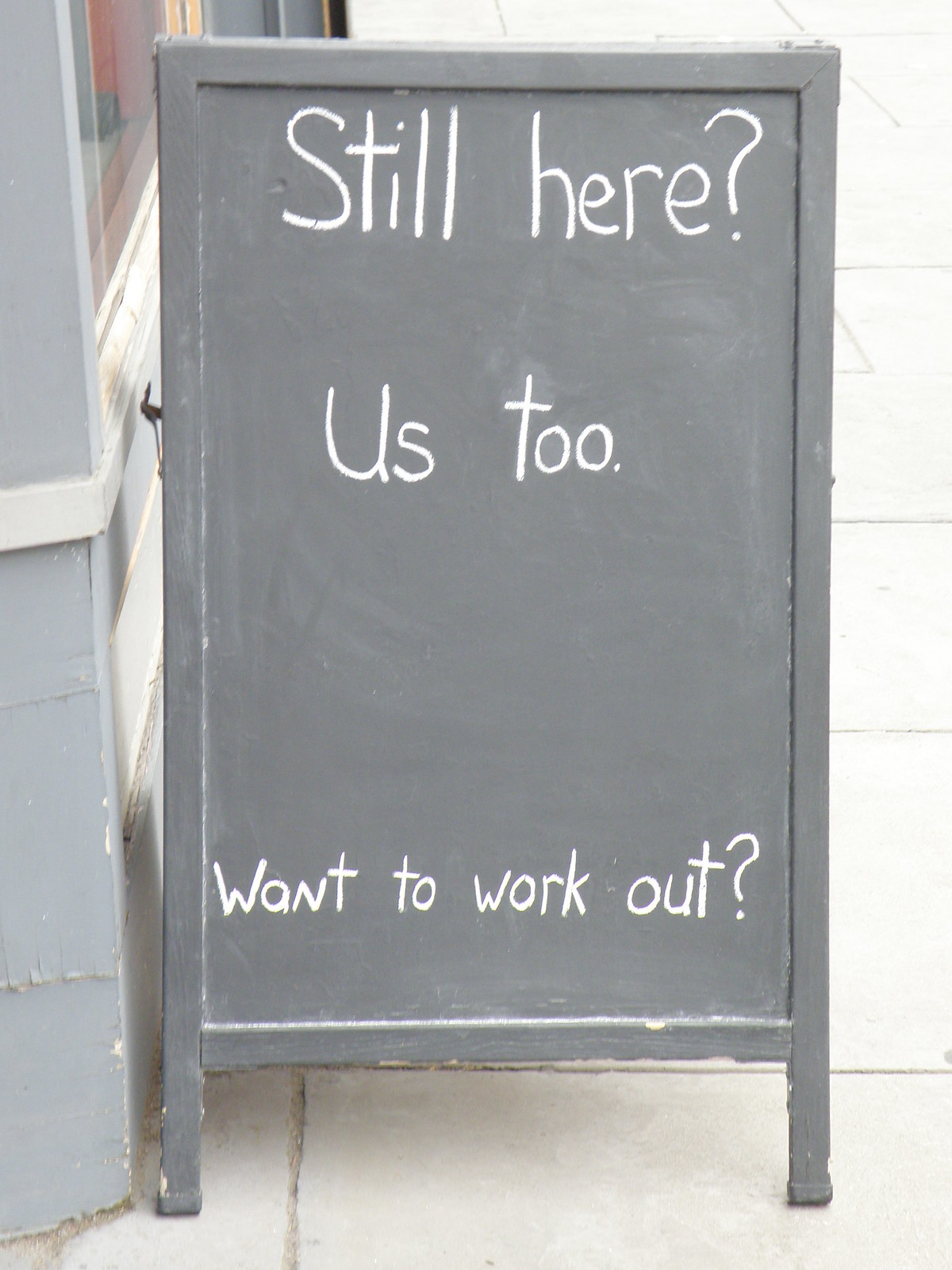The image captures a scene set on a cement sidewalk with a light grey brick pattern. Centrally featured is a dark grey, fold-out chalkboard sign positioned in front of a greyish-blue building on its left. A window on the building is partially visible, and the scene is bathed in daylight, with a shadow cast by the sign to the left, suggesting sunlight coming from the right.

The sign itself has a somewhat dusty and aged appearance, indicative of its longtime use. Written in white chalk in a spread-out hand-lettered style, the sign reads: "Still here? Us too. Want to work out?" The humorous message, coupled with the question about working out, strongly suggests it is placed outside a gym trying to attract potential clients to come in and exercise. The overall ambiance combines a touch of humor with a welcoming invite for passersby to consider working out at this establishment.